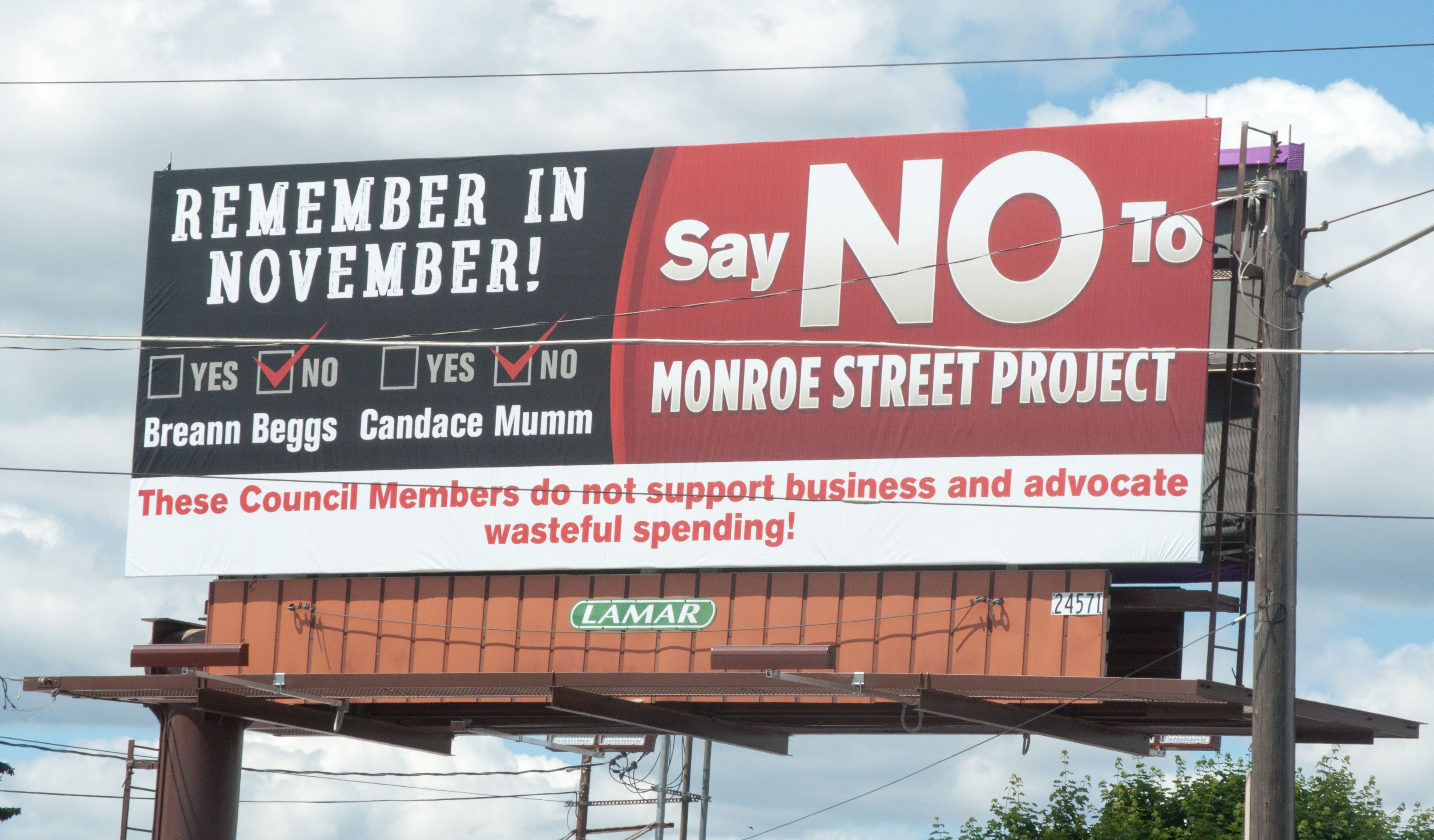This image captures a daytime photograph of a large, prominently placed billboard against a backdrop of a blue sky and fluffy clouds, intended for city drivers. The billboard features the text "Remember in November" in bold letters. Below this, two names are listed: Breanne Beggs and Candace Mumm, each accompanied by a checkbox marked "NO." To the right, in a red section that splits the board, it reads, "Say NO to Monroe Street Project." At the bottom, on a white runner with red lettering, the text states, "These council members do not support business and advocate wasteful spending." The billboard is mounted on a structure labeled "Lamar," bearing the identification number 24571. The imagery and messaging emphasize a call to action, urging the public to vote "NO" and oppose the Monroe Street Project.